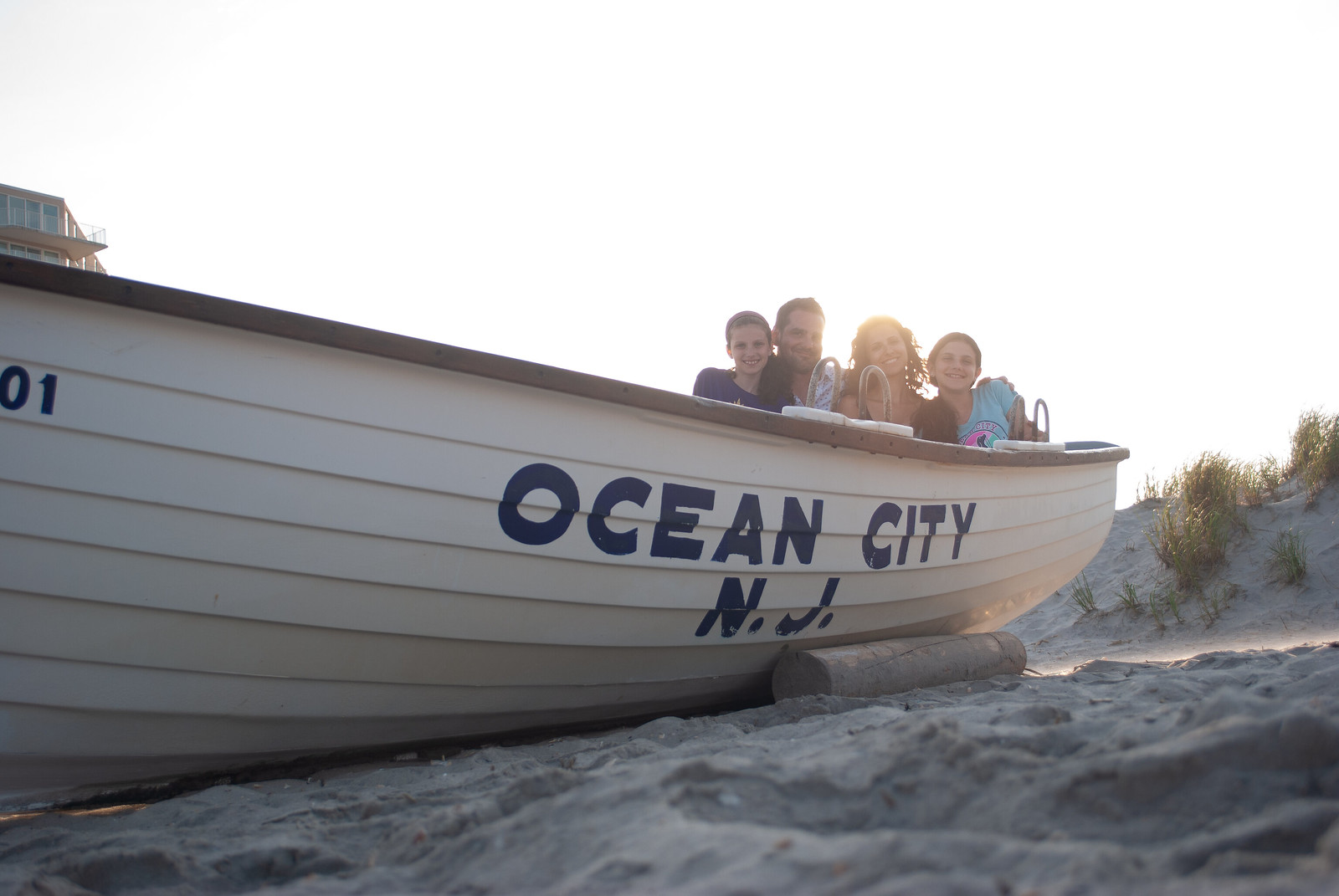In this outdoor beach scene, a camera captures a low-angle shot from sand level, focusing on a cream-colored boat situated on the sandy shore. The boat, sporting blue text reading "Ocean City, New Jersey" along with the number '01,' serves as a picturesque prop for a family portrait. Seated in the boat are a mother, a father, and two young girls, all smiling brightly at the camera. Behind them, a sand dune dotted with green tufts of grass rises in the background, adding a natural element to the setting. Notably, a log placed under the boat keeps it steady, and the sky suggests the sun may be setting, casting a warm glow over this serene and joyful moment.